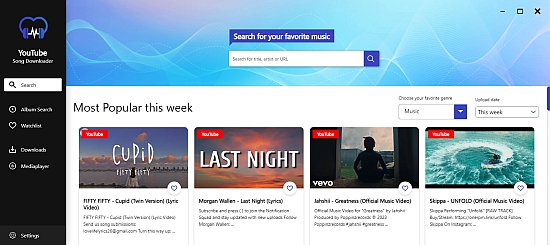The screenshot showcases the interface of a software application titled "YouTube Song Downloader." Dominating the top left section is a logo featuring a heart shape seamlessly merging into headphone cups, with a stylized sound wave connecting the two sides. Beneath this logo, the left-hand menu, set against a black background, includes several options: a searchable field, followed by "Album Search," "Watch List," "Downloads," and what appears to be "Media Player." Unfortunately, the text is too small to be certain. At the very bottom of this menu is a settings icon represented by a cogwheel.

The header of the interface displays simple, wavy blue computer graphics. Right below it is a rectangular speech bubble prompting, "Search for your favorite music," with an adjacent search field that can be used to search by name or URL. 

Below this search field is a section titled "Most Popular This Week," which lists trending songs: "Cupid" by an artist whose name could not be clearly discerned, but the initials appear to be "Hitty Fitty" or "Itty Nitty," available on YouTube. Other popular titles include "Last Night" by Morgan Wallen, also on YouTube, and several other unnamed tracks. Depicted within the interface is an image of someone riding a jet ski in the ocean, hinting that users can download videos or audio directly from YouTube using the application.